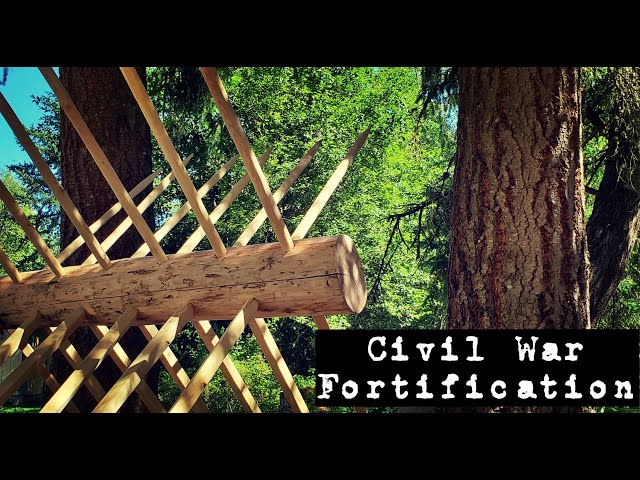In the image, there's a notable black framing comprising thick black rectangles at the top and bottom. The primary focus of the picture is an outdoor scene set in a field surrounded by a forest with large, dark-brown tree trunks. Centrally visible is a wooden structure—likely a wartime trap or fortification—made from a log embedded with numerous spikes and sticks, arranged as if it could swing from a tree. This setup, reminiscent of Civil War fortifications, adds a historic context to the image. Prominently, in the lower right corner, a black rectangle contains white text that reads "Civil War Fortification," further emphasizing the historical significance of the depicted wooden weaponry. The overall backdrop appears bright, suggestive of clear daylight conditions.